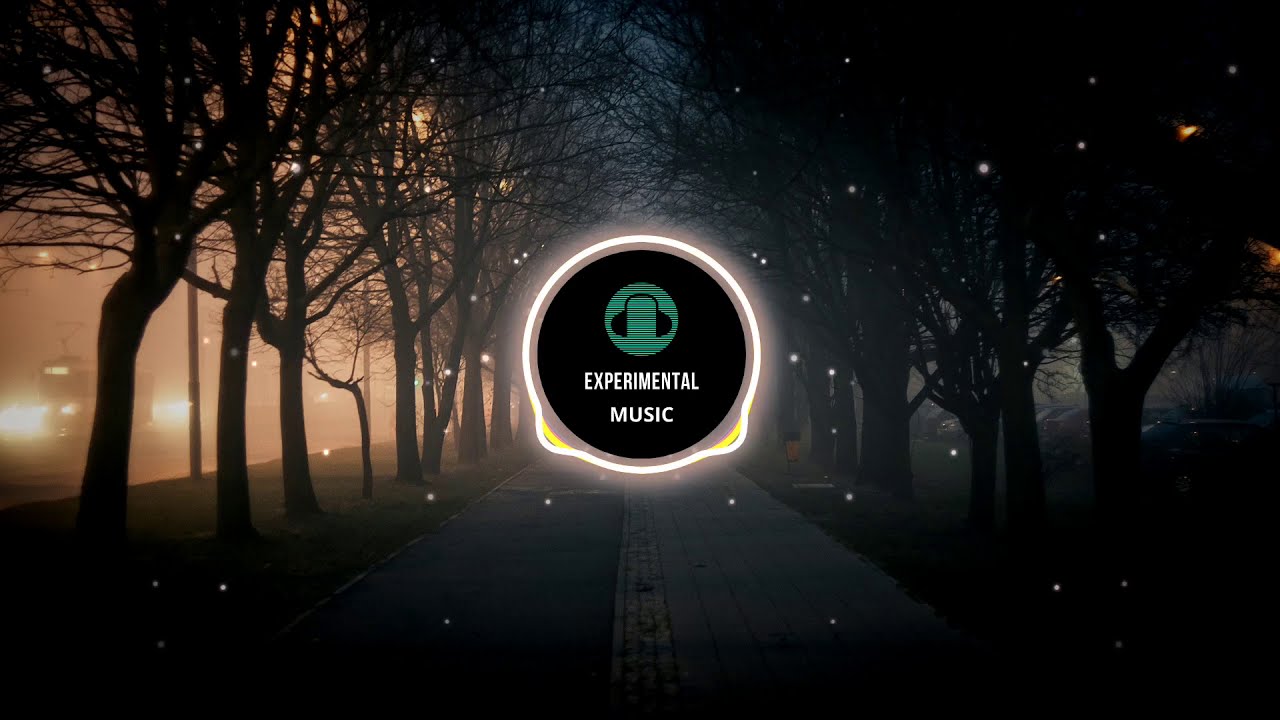The image is a dark, horizontal rectangle that appears to be a screenshot from a YouTube music video or possibly a music program or video game. The scene depicts a park setting during the evening, with trees flanking both sides of a central road or sidewalk. On the left side, street lights or vehicle headlights create a foggy appearance, and there's a vehicle, possibly a bus or electric cart, moving down the road. The right side also shows more trees and parked cars. The sky is a very dark blue, indicating it is evening. 

In the center of the image, there's a prominent circular logo that features a pair of headphones inside a green circle. This green circle is encircled by a larger black circle, which is then outlined by a bright white circle. The words "EXPERIMENTAL MUSIC" are prominently displayed in white, all-caps letters against the black circle. Scattered white dots resembling stars are sprinkled across the image, adding to the dark, serene atmosphere.